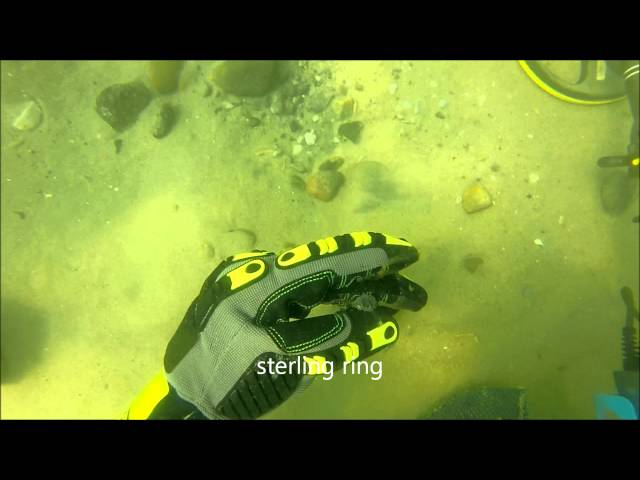In this underwater image, the left hand of a scuba diver, donned in a distinctive glove with black and yellow stripes on the fingers and black stitching on the inside, is prominently displayed. The glove itself is gray, and the diver is holding a sterling ring between the middle finger and thumb. The scene is set at the bottom of a body of water, where rocks can be seen above the hand, curving to the right. In the upper left corner of the image, a metal detector is partially visible, with just enough of the ring and part of the stem showing to identify it. The glove is centrally positioned, making it the main focus amidst the rocky underwater surroundings.